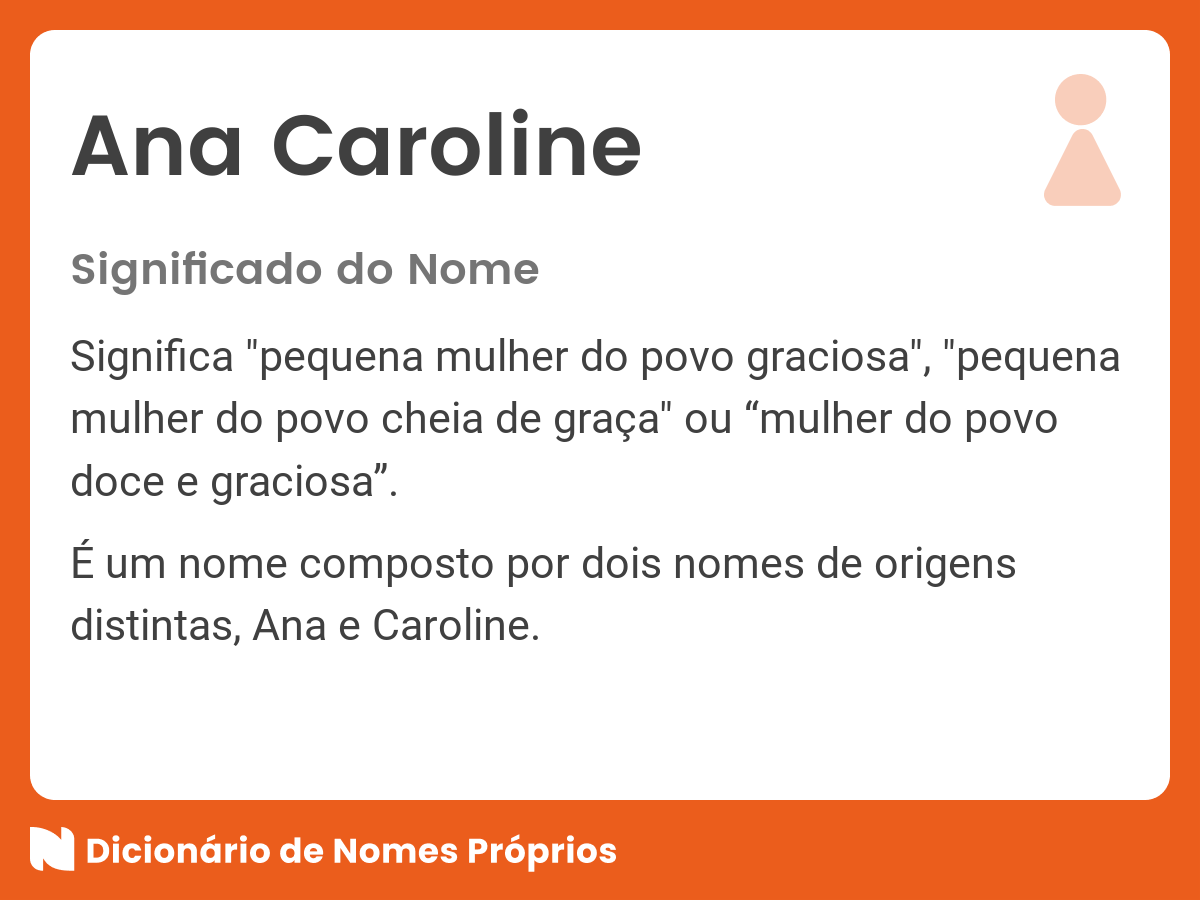The image depicts a card with an orange border, which is thicker at the bottom and thinner around the rest. The center of the card features a white background with black lettering prominently displaying the name "Anna Caroline." To the right of the name, there is a light pink symbol resembling a circle resting on a triangle, possibly representing a female figure. Below this, in black text, is Spanish content explaining the meaning of the name "Anna Caroline," describing it as "significado do nome, significa pequena mulher do povo gracioso," which translates to a small, graceful woman of the people. The description also mentions that it is a compound name comprising "Anna" and "Caroline," each with distinct origins. At the very bottom of the card, within the thick orange part, there is a logo featuring the letter "N" and the phrase "Diccionario de Nombres Propios" in white font.